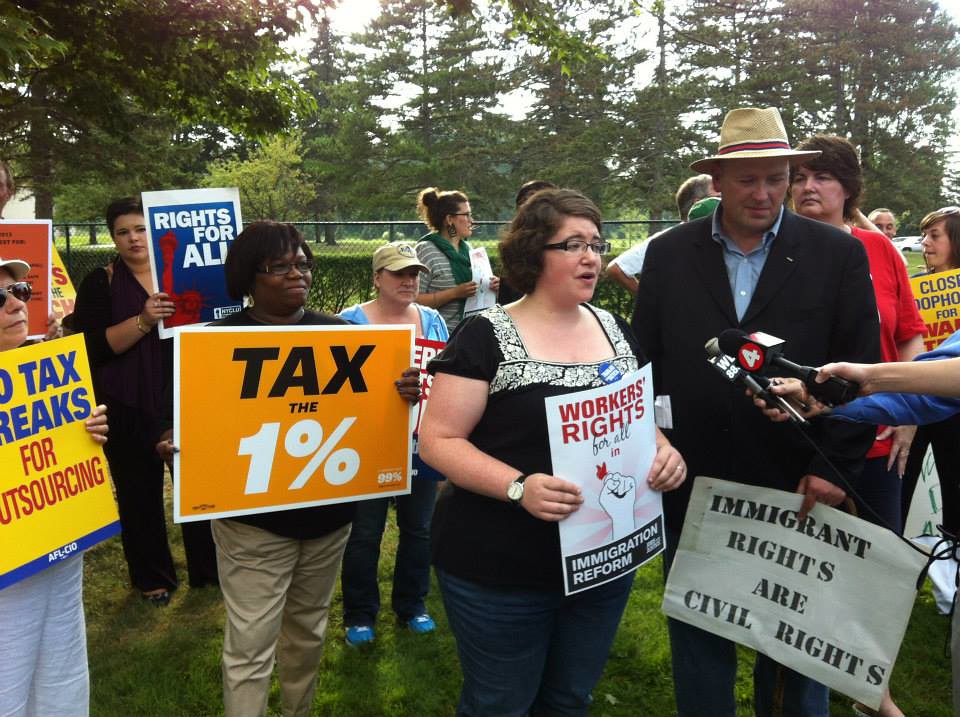The image depicts an outdoor daytime demonstration in a park-like setting, with grass underfoot and tall pine trees in the background, along with a chain-link fence. Prominently featured are two microphones held before a group of protesters, one microphone labeled with a red circle that reads "Channel 4" and the other obscured but with white lettering. The diverse crowd includes people from various ethnicities, all holding signs advocating for different causes.

At the forefront is a short-haired Caucasian woman, noticeably overweight, dressed in a black top, blue jeans, and black glasses. Her sign demands "Workers' Rights for All" and calls for "Immigration Reform," illustrated with a raised fist on a red background. Beside her stands a man in a black suit with a light blue denim shirt and a tan hat. He grasps a white sign declaring "Immigrant Rights Are Civil Rights."

In the background, a Black woman holds up a gold sign stating "Tax the 1%." Nearby is a Latino woman with a sign that reads "Rights for All," set against a blue background. Another partially visible sign hints at the phrase "Tax Breaks for Outsourcing" but is cut off. The scene captures the energy and diversity of the protest, highlighting various social justice issues in a unified call for change.